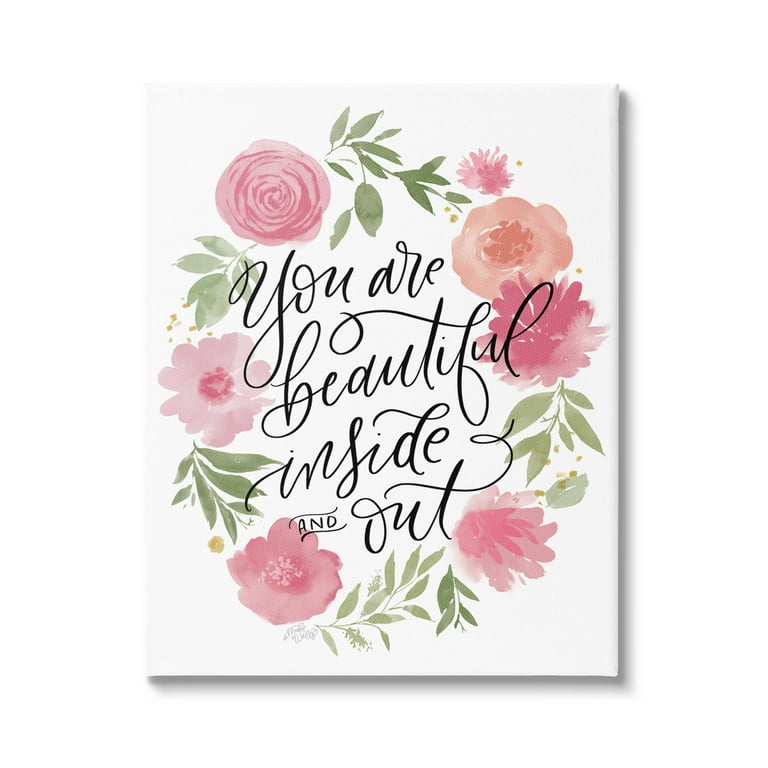The image is a color illustration with typography, designed as a wall art piece in portrait orientation. It features a white canvas on a white background, casting a soft shadow towards the lower right, suggesting light from the upper left. Encircling the canvas text is a vertical elliptical garland of watercolor-effect flowers and leaves. The floral ring includes blossoms in shades of pink and peach, interspersed with green leaves. At the center, the text, handwritten or in a custom script font, reads, "You are beautiful inside and out." The phrase is slightly angled, with the word "and" appearing in a tiny size flanked by two squiggly lines above and below. The overall style combines illustration and typography to deliver an inspirational message, perfect for wall decor.